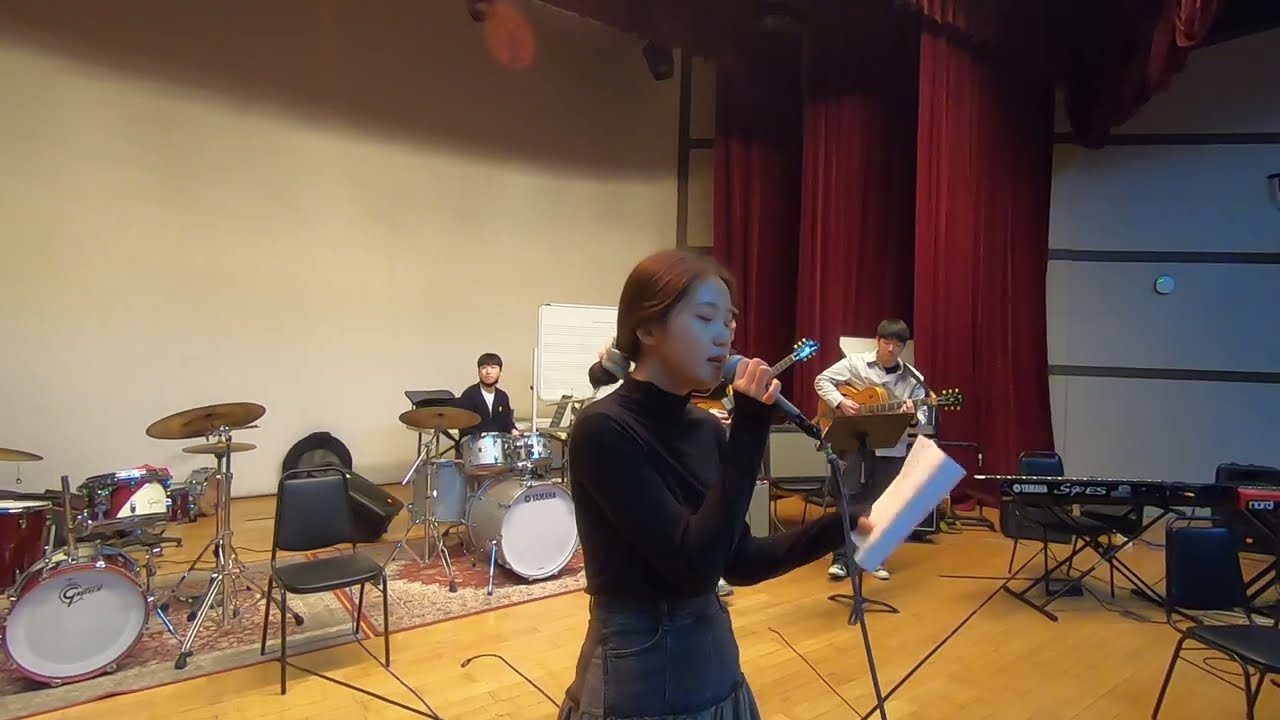This image captures a detailed scene of a musical practice session on a stage with wooden flooring. The focal point is a young Asian woman standing front and center, holding a microphone in one hand and a notebook with lyrics in the other. She is dressed in a black shirt and is looking to her right. Directly behind her is a beige wall with a whiteboard, and over her right shoulder sits a drummer at a red Gresh drum set. To the drummer's left is an open black chair and an unoccupied silver Yamaha drum set. Over the woman's left shoulder is a guitarist in a light brown shirt, with red curtains in the background. To the right of the guitarist is a keyboard positioned near more scattered black chairs. The stage is completed with two rugs under the drum sets, displaying a tan and red pattern. The overall setting, adorned with classical red curtains and situated in what appears to be a large auditorium, suggests a rehearsal in a music school, strongly hinting at a Japanese origin due to visible Japanese writing on the back wall.